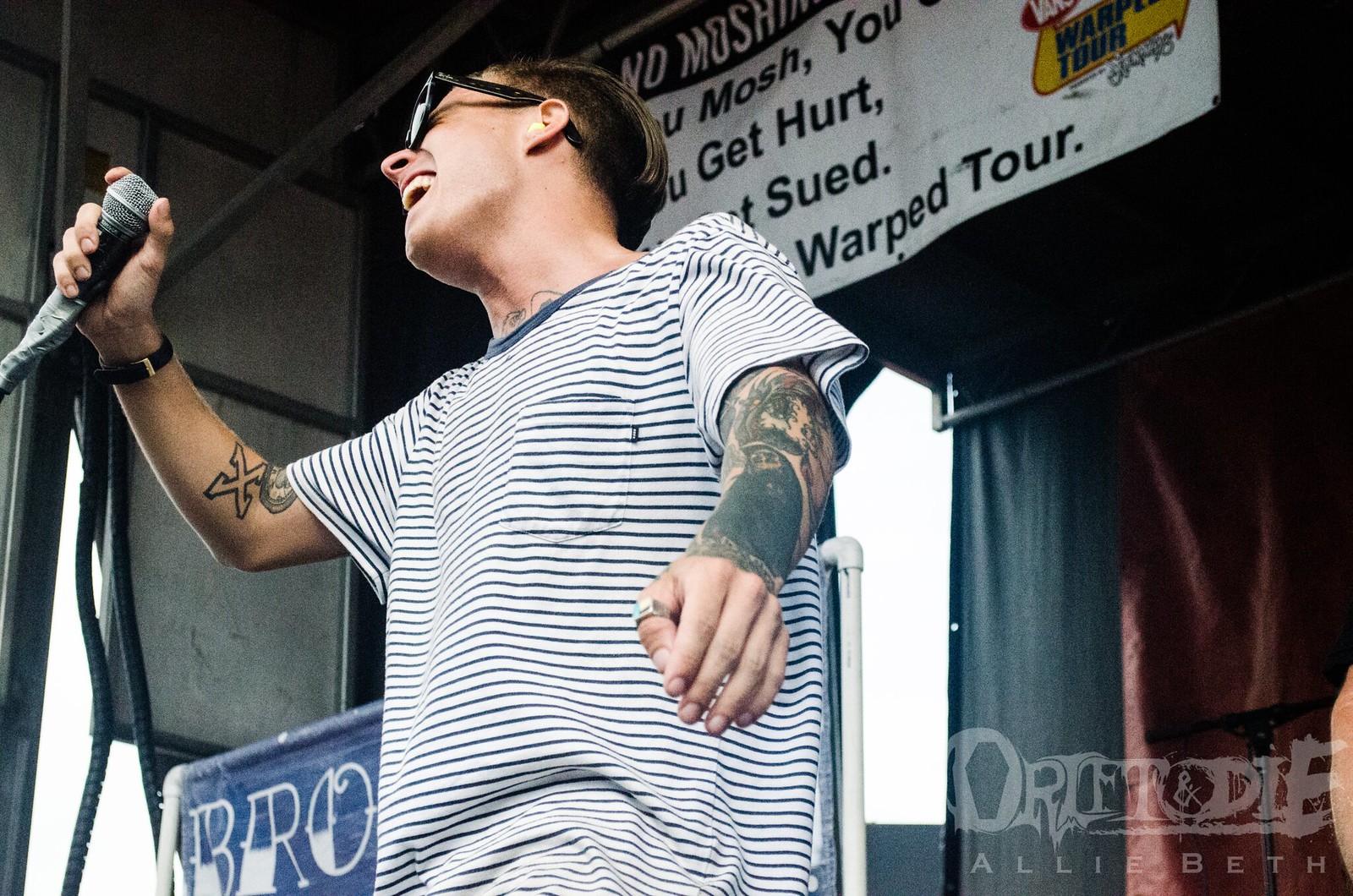In this photograph, a younger man stands center stage, captured from a low perspective that accentuates his presence. He holds a microphone with his right hand, his arm bent at the elbow, displaying a prominent X tattoo. His left arm extends towards the center of the image, revealing numerous tattoos and a watch band. He wears a white shirt with blue horizontal stripes, dark glasses, and his dark hair frames an open mouth, suggesting he's either singing or speaking into the microphone. Above him, a white sign hangs from the ceiling with the partially visible text: "No moshing. You mosh, you get hurt." The stage setup includes a blue drape and visible scaffolding, framed against a backdrop of what might be an open space or window. Red curtains hang behind him, adding an element of drama. In the bottom right corner, white text reads, "Orff, Toadie, Allie, Beth."